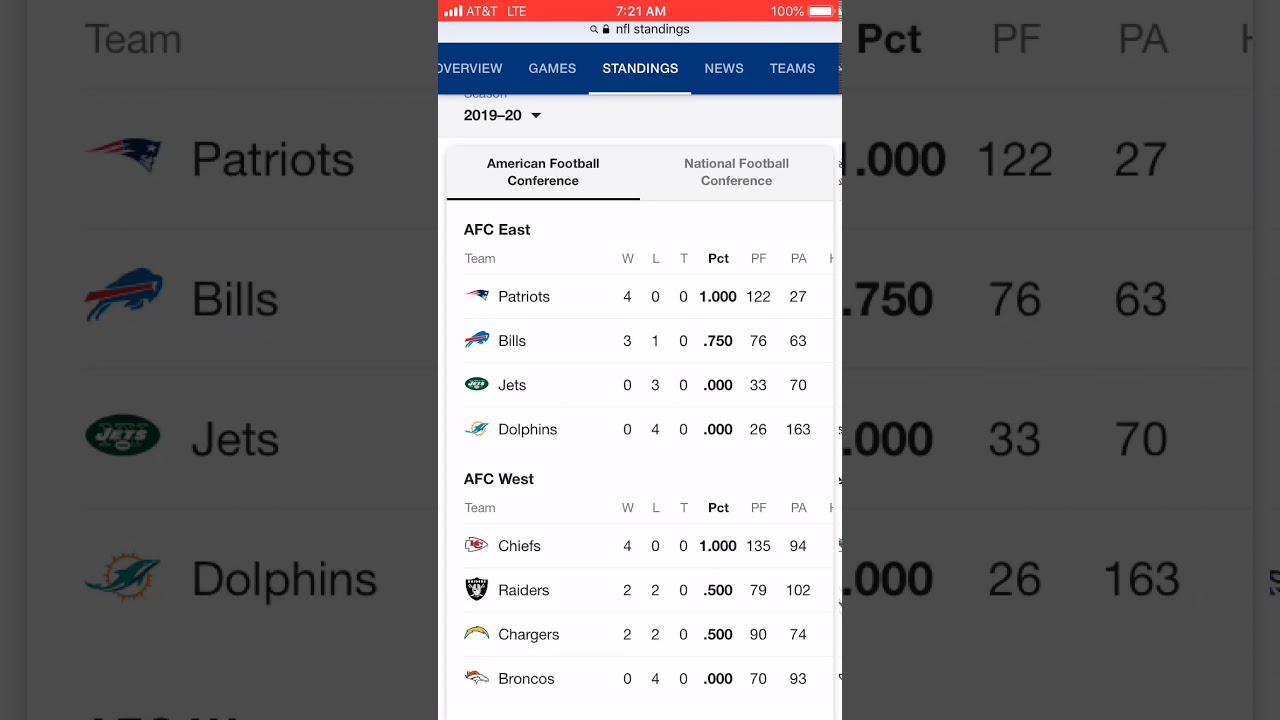This screenshot captures a detailed view of NFL standings, prominently featuring a layered interface. In the backdrop, grayed out, you can discern football statistics and team logos. These logos include the New England Patriots with their iconic red, white, and blue head symbol; the Buffalo Bills with a blue and red buffalo; the New York Jets in green and white; and the Miami Dolphins with a blue dolphin. Text such as PCT, PF, PA denotes percentage, points for, and points against, respectively.

Overlaying this background is an active window with distinct elements. At the top, a red bar displays the status indicators: AT&T LTE for network, signal strength bars, the current time "7:21 AM", and a battery status showing 100% charge.

Below this bar, the window header reads "NFL standings" accompanied by a black padlock icon for security and a magnifying glass for search functionality. The interface features a blue section with submenus labeled "Overview", "Games", "Standings" (highlighted in white with an underscore), "News", and "Teams."

Further down, the years "2019" and "2020" are marked, transitioning to the conference breakdown. The "American Football Conference (AFC) East" lists teams and their logos: Patriots, Bills, Jets, and Dolphins. Similarly, the "AFC West" section lists the Kansas City Chiefs with their arrowhead logo, the Las Vegas Raiders with a black and white pirate, the Los Angeles Chargers with a gold lightning bolt, and the Denver Broncos with an orange and white horse.

Each team is associated with various statistical categories, listed as WLT (win-loss-tie), PCT (percentage), PF (points for), and PA (points against), showcasing their performance metrics.